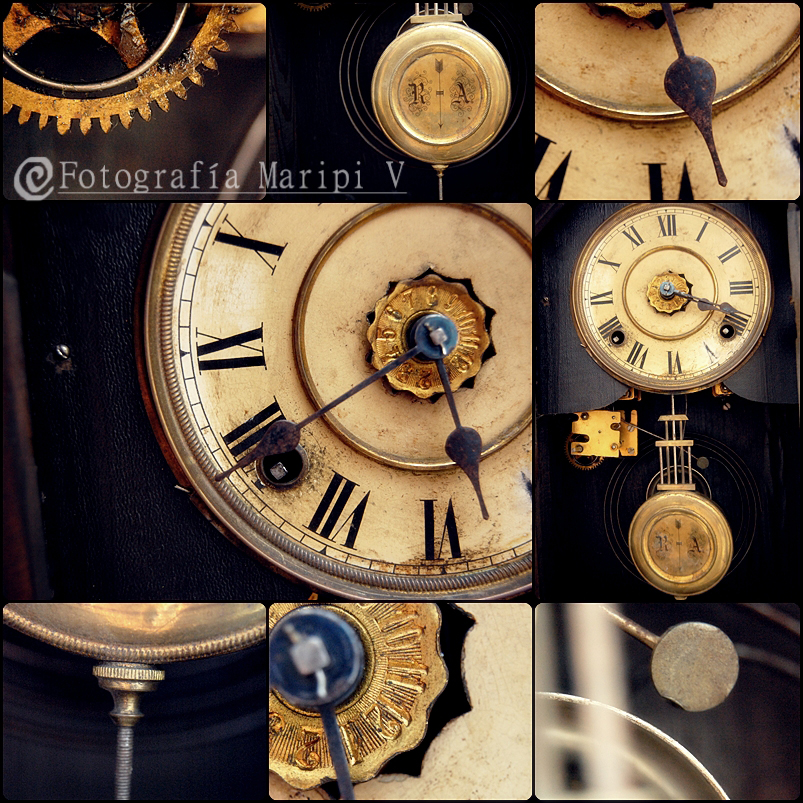This detailed photo collage features a collection of clocks, predominantly showcasing clock faces adorned with Roman numerals. The centerpiece is a clock where the hour hand rests between the V (five) and VI (six) marks, while the minute hand points directly at the VII (seven). The clock's hands are anchored by a striking blue piece, set against a gold backdrop. Above the collage, the social media handle "Photographia Maripi V" is prominently displayed, underlined for emphasis. Notably, there is a deliberate space between "Photographia," "Maripi," and "V," making the profile name stand out distinctively.